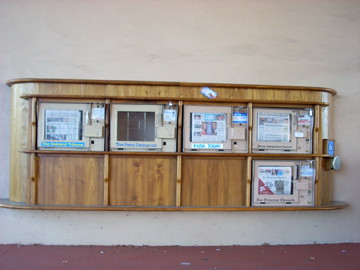The image depicts a wooden newspaper dispenser with a distinctive design featuring a curved edge and a long straight surface, attached to a wall. The dispenser is subdivided into sections for five different newspapers, identified by their front-page images. Four sections are positioned across the top of the structure, each with a coin slot for inserting money to purchase a newspaper, while the fifth section, slightly elevated, appears empty. Notably, a wheelchair accessibility button is visible on the right side of the dispenser, which might aid in opening the coin-operated slots automatically. The entire setup, evoking an old-fashioned yet functional charm, rests slightly above ground level, creating a unique, eye-catching kiosk-like appearance.